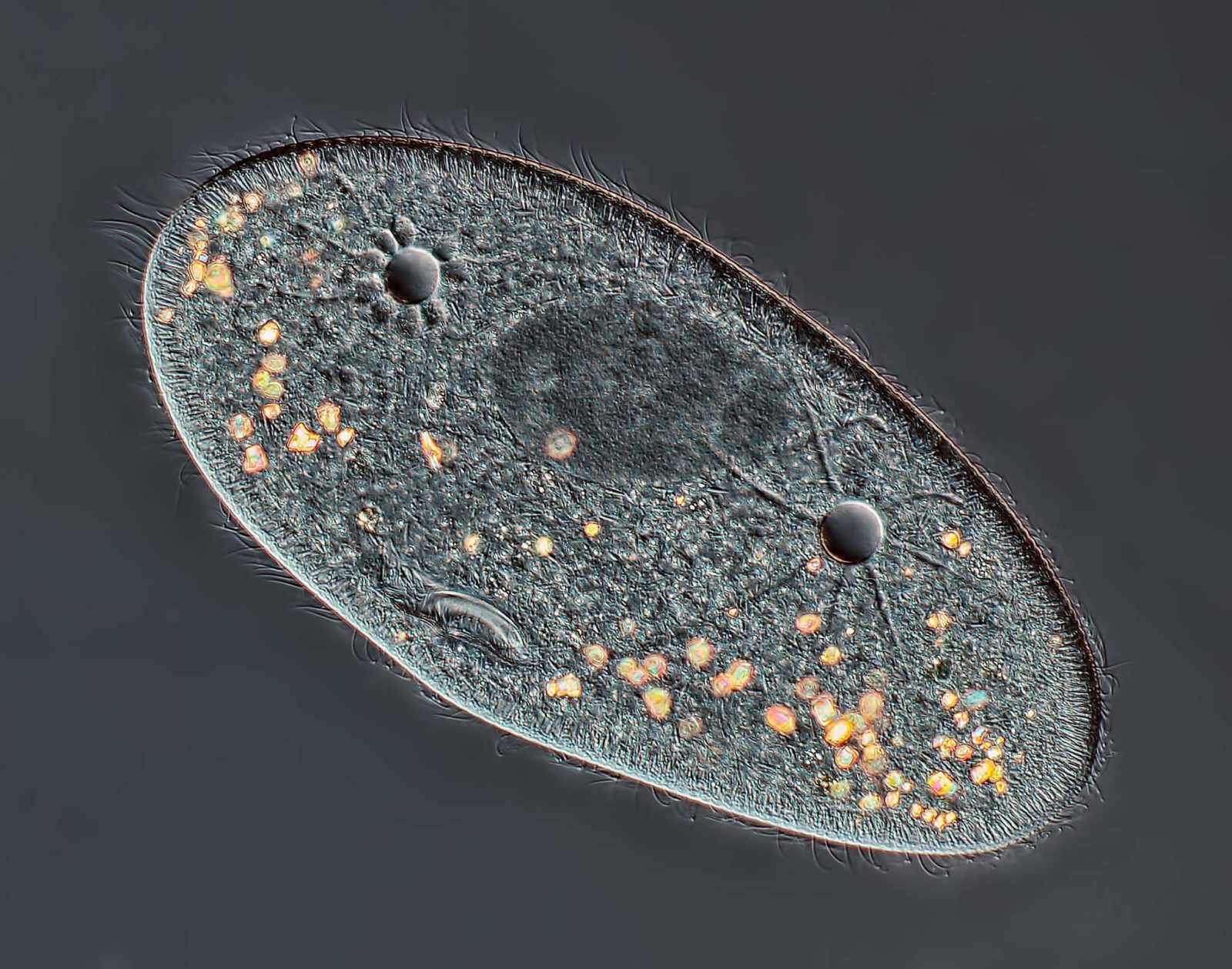This detailed microscopic image showcases a single-celled organism, possibly an amoeba or a bacterium. It dominates a gray background with its elongated, oval shape, oriented toward the bottom right corner. The cell's exterior displays a pinkish hue with hair-like flagella emerging from its surface, giving it a furry appearance. The interior is filled with a gray, gel-like material and features distinct structures: a prominent dark spot near the top center, flanked by two smaller black circles. There are also black circles with radial lines, reminiscent of a suns, further down the cell. Scattered across its surface are numerous glowing orange-yellow spots, particularly concentrated towards the bottom. The organism's overall coloration includes shades of blue and sporadic yellowish-gold spots, contributing to a vibrant and complex visual structure.